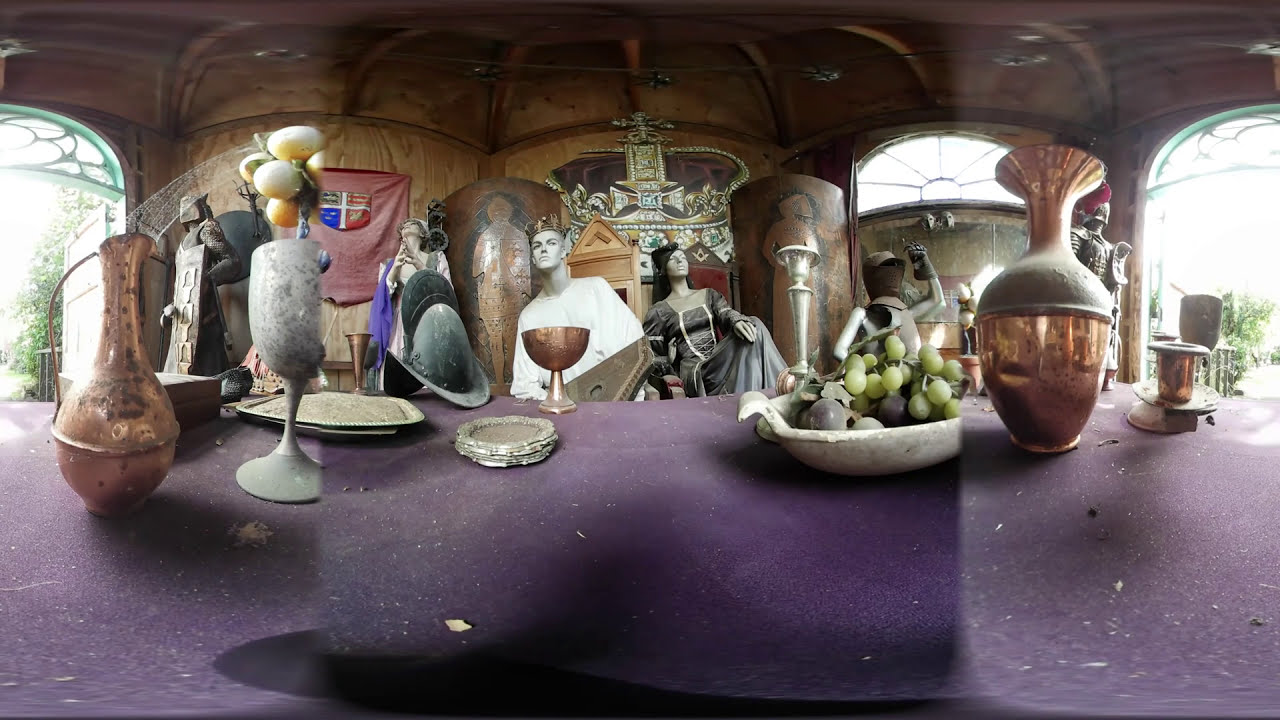This highly detailed and surreal photograph appears to capture a meticulously designed medieval set, possibly for a play or an artistic installation. The centerpiece is a lavish purple table, arrayed with an eclectic assortment of historic-looking goblets, chalices, vases, and copper pitchers. A bowl of green grapes adds a touch of color and organic texture. Surrounding the table are mannequins staged in royal thrones, evoking a sense of ancient majesty. A gray, bald male mannequin is adorned in a white shirt, while a female mannequin beside him wears an elaborate, gray silk gown with silver accents, reminiscent of medieval royalty. The backdrop features more mannequins, some clad in knightly armor, adding to the historical ambiance. This scene is framed by a structure that could be an open gazebo or an indoors wooden setting with light streaming through cut-out arcs or windows. Additional elements like a shield with a coat of arms, a hanging flag with red and blue hues, statues, and scattered paintings enhance the intricate detailing and complete the medieval tableau. The dominant colors in this striking image include shades of copper, gold, yellow, black, white, gray, brown, red, green, pink, and silver.